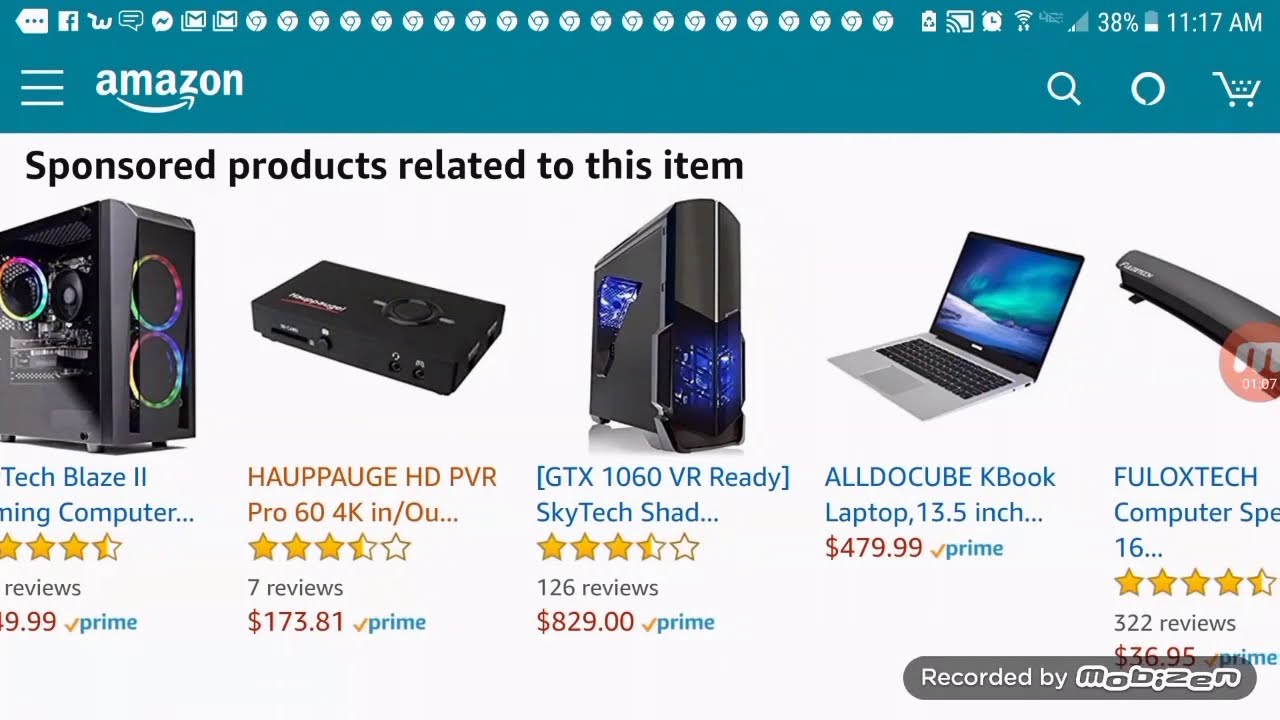The screenshot displays a cropped close-up of an Amazon page on a mobile device. At the top, a teal-blue header features several elements. On the left, three horizontal white lines represent the menu icon. Adjacent to this is the Amazon logo, which includes an arrow curving upward to the right. Toward the right-hand side of the header are three white icons positioned from left to right: a magnifying glass, a circle, and a shopping cart.

In the notification bar above the header, multiple notifications and status icons are present. From left to right, there is a tag with three blue dots pointing left, a white square with a blue "F" (likely a Facebook notification), a white "W" with a flange on the left, a white message box, a white speech bubble with a blue horizontal lightning bolt, two stacked envelope icons, and numerous white Chrome icons depicting a white circle with a blue center and three blue lines radiating outward. At the far right, additional status indicators include a white battery logo showing 38% charge, a white casting-to-screen icon, a white clock, a Wi-Fi logo, two out of five mobile data bars, and the time, 11:17 AM.

Below the teal-blue header, the page features a white background displaying the text "Sponsored products related to this item." Below this, several computer-related items are showcased, each accompanied by a name, price, number of reviews, and star rating. In the bottom right corner of the screen, a watermark with a gray background and rounded edges contains white text reading "Recorded by Mobizen."